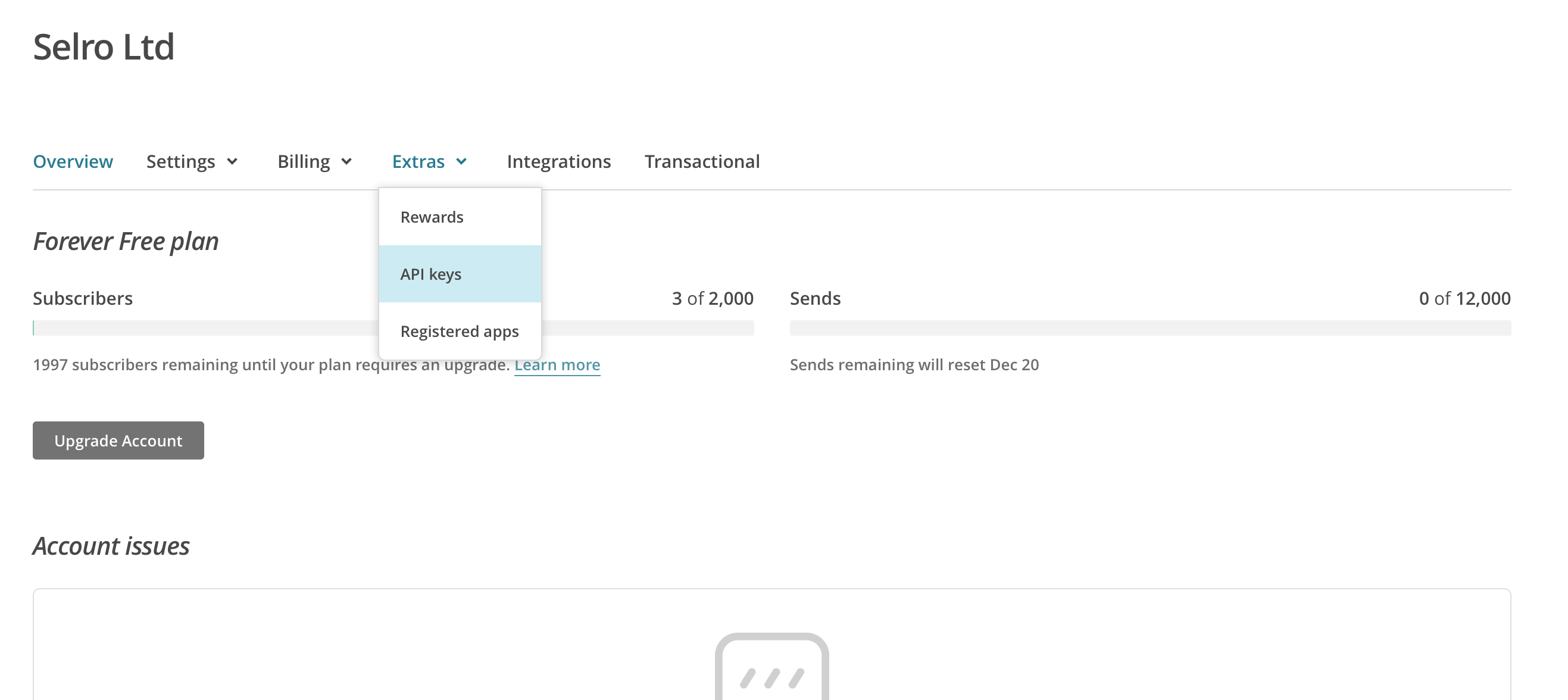This is a cropped screenshot of a Selro LTD inventory and order management platform user interface. At the top left corner, "Selro LTD" is prominently displayed in bold black font on a white background. Just below, a horizontal menu bar features several categories: "Overview," "Settings," "Billing," "Extras," "Integrations," and "Transactional." Both "Overview" and "Extras" are highlighted in blue, indicating selected sections. A drop-down menu under "Extras" lists "Rewards," "API Keys," and "Registered Apps," with "API Keys" highlighted in blue, indicating it is the current selection.

On the lower left, the text "Forever Free Plan" is shown in bold, black italicized font. Beneath this heading, a progress bar labeled "Subscribers" displays in graphical form that 3 out of 2,000 subscriber slots are used. The right side of the progress bar indicates "1,997 subscribers remaining until your plan requires an upgrade," with a "Learn More" option available as a blue hyperlink. Below this, a gray button labeled "Upgrade Account" provides an option for account enhancement.

On the right side of the page, the word "Sends" appears in small black font above another progress bar. Above this bar, numerical values show "0 of 12,000" sends utilized. Beneath the bar, it is noted that "Sends remaining will reset December 20th."

At the bottom left, the text "Account Issues" appears in black italicized font. The screenshot is carefully cropped, ensuring all essential information is contained within the borders of the image.